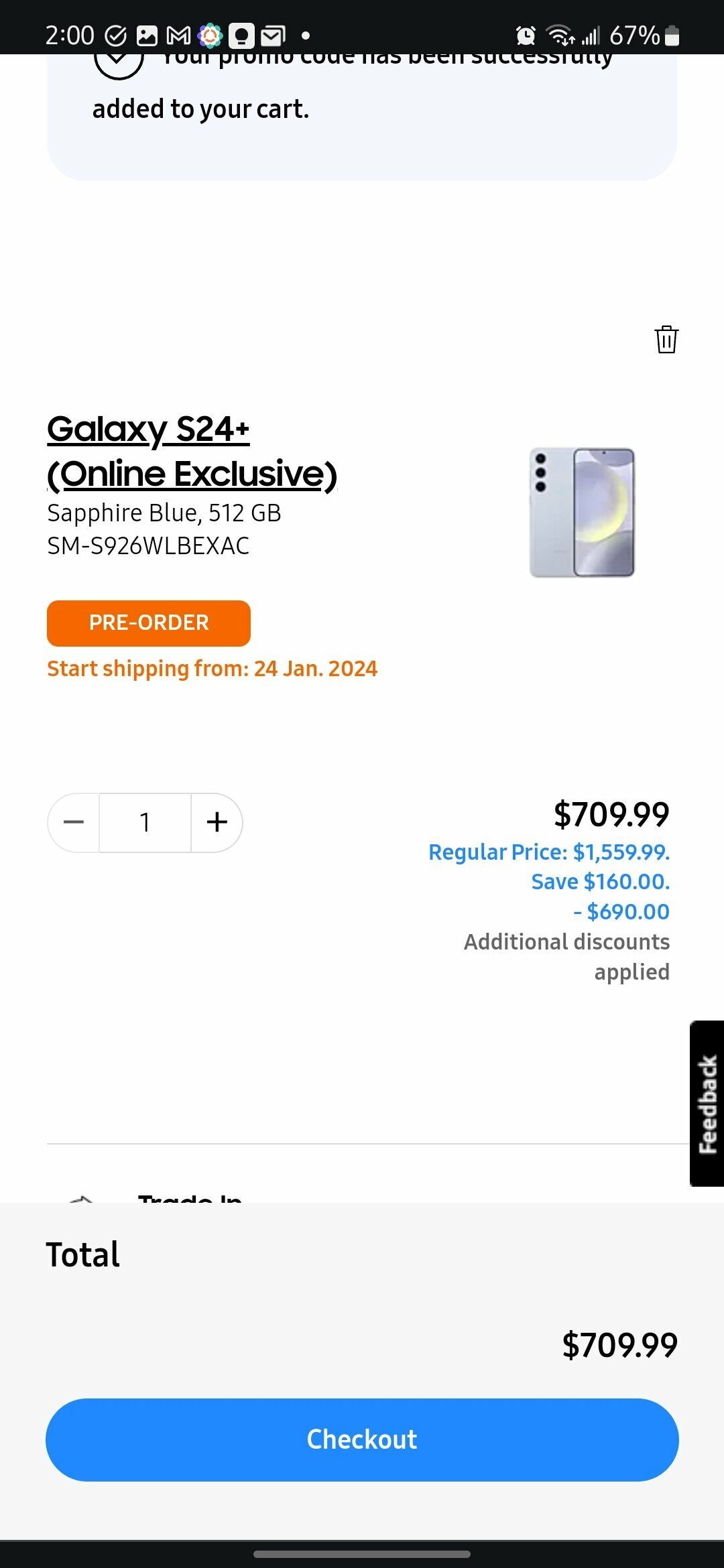The image showcases an online shopping cart on a mobile device, in which an individual is about to purchase a Galaxy S24+ smartphone. The smartphone is an online exclusive and includes 512GB of storage. It is offered in a striking sapphire blue color, and it is available for pre-order, with shipments expected to start on January 24, 2024. At the top of the image, the mobile phone's taskbar is visible, displaying the current time, battery percentage, Wi-Fi connection status, and open notifications.

On the actual shopping cart page, there is one Galaxy S24+ phone listed, with a marked quantity of one. The current price listed for the phone is $709.99. Highlighted in blue text below this is the regular retail price, which is $1,559.99, indicating that the buyer is saving a total of $850, thanks to a discount of $690 plus an additional $160 discount.

At the bottom of the screen, the total cost is reiterated in bold black text, clearly showing the final amount as $709.99. The page also features a prominent blue "Checkout" button, urging the user to complete their purchase.